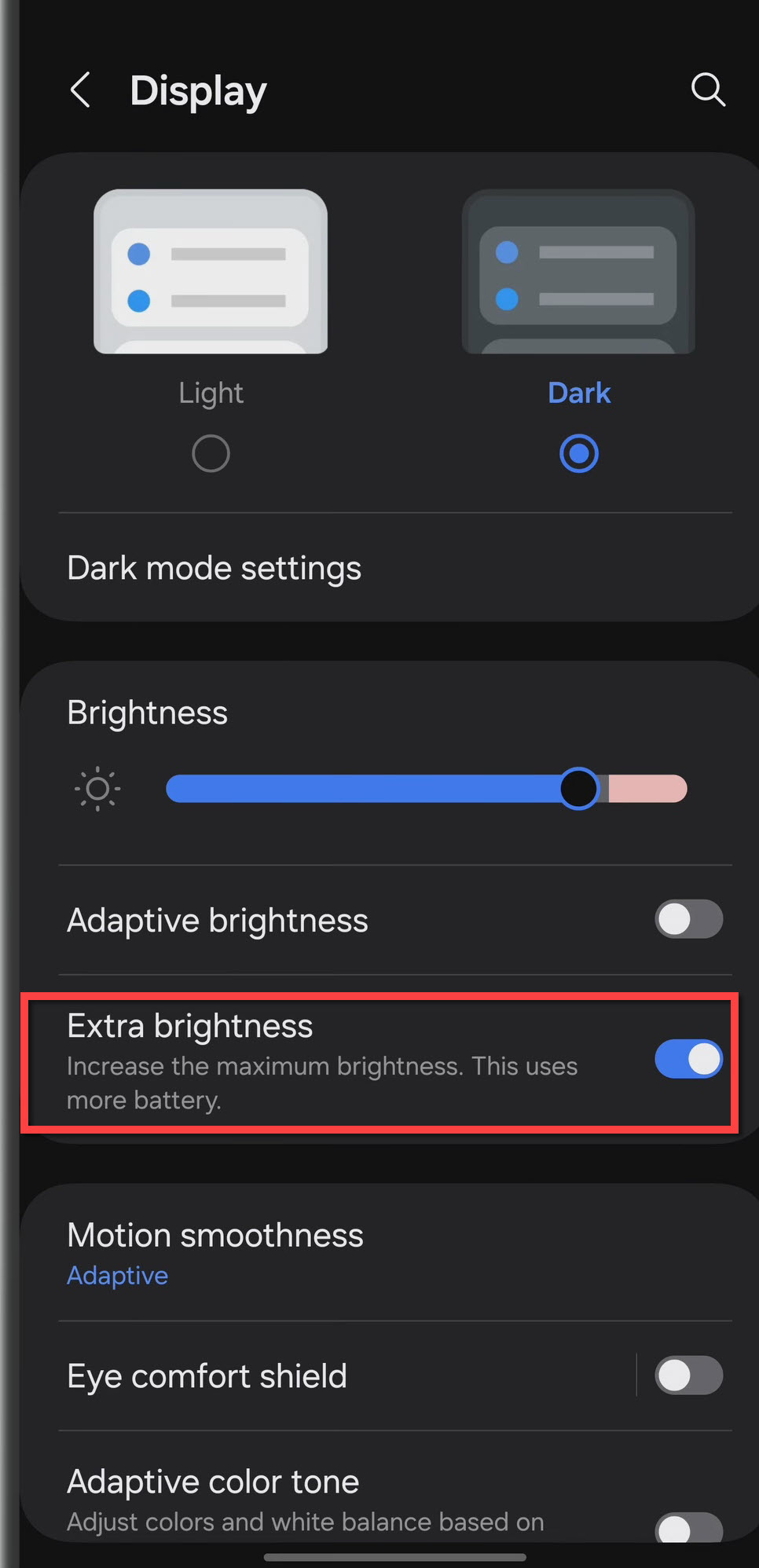**Detailed Caption:**

This image displays the settings menu of a smartphone in Night Mode, characterized by a black background and white text. At the top left, the heading "Display" is prominently featured. Below this heading, the screen is divided into two sections: "Light Mode" on the left and "Dark Mode" on the right. The "Dark Mode" option is highlighted in blue, indicating that it is currently selected.

Beneath these sections, on the left side, is the text "Dark Mode Settings," followed by "Brightness." Adjacent to the "Brightness" section, there's a blue brightness slider with a movable black circle. The slider is positioned nearly to the right, suggesting almost maximum brightness, with an additional shaded pink level that exceeds maximum brightness.

Further down, the text "Adaptive Brightness" is shown, accompanied by a toggle switch that is off, indicated by its gray color. Below this, the caption reads "Extra Brightness" with the subtext "Increase the maximum brightness, this uses more battery." The toggle for "Extra Brightness" is on, as shown by its blue color, and it has a red outline to highlight this selection.

Continuing down, the caption mentions "Motion Smoothness" set to "Adaptive," with the term "Adaptive" written in blue while the rest of the text remains white. Below that, "Eye comfort shield" is listed, with its toggle switch turned off, evidenced by its gray color. Finally, the "Adaptive Color Tone" feature is described as adjusting colors based on white balance. This feature is also turned off, as indicated by the gray toggle switch.